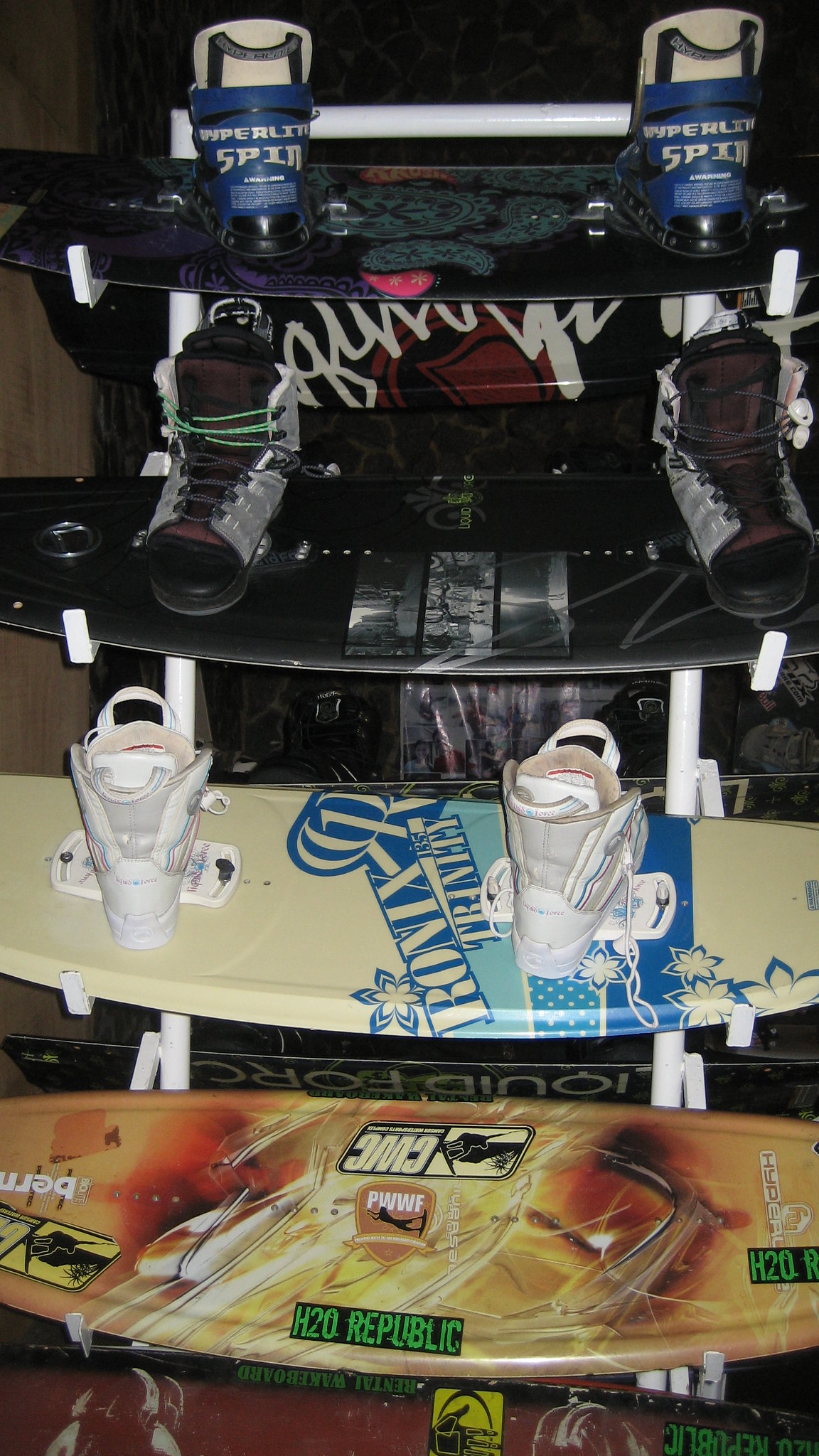The image showcases a display case within a shop, possibly a second-hand sporting goods store, ski shop, or winter gear rental place, featuring a unique shelving arrangement made from four snowboards or skateboards, each positioned one atop another within a sleek, white powder-coated frame. The topmost shelf holds blue snowboard boots with an indistinct logo on a black board adorned with a green insignia. Below, the second shelf features black and gray boots with burgundy accents, matching a black and gray board. The third shelf exhibits white boots on an off-white and blue board. The bottom shelf, devoid of footwear, displays a brown and yellow board with pre-drilled holes for potential attachments. Each board creatively acts as a shelf to not only display different types of sporting footwear but also suggest a cohesive aesthetic where the color schemes of the boots and boards are harmonized, possibly hinting at the best gear combinations for snowboarding enthusiasts.